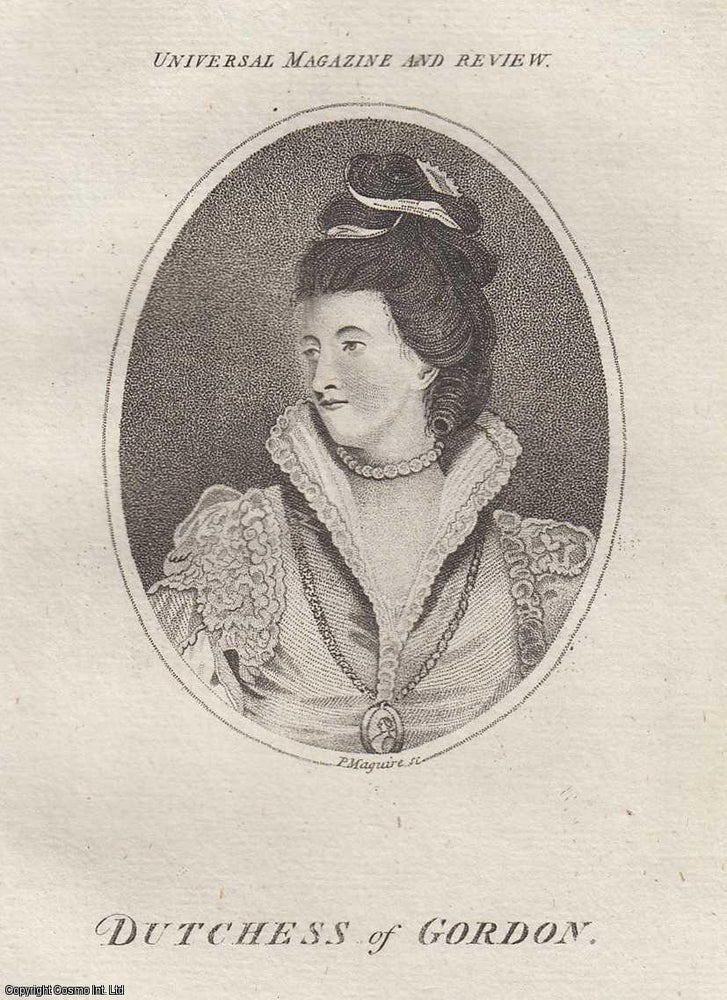The image is a rectangular, six-inch tall by three-to-four inch wide old print from Universal Magazine and Review, featuring an oval tintype photograph of the Duchess of Gordon, likely from the 1800s. The background is an off-white hue, evocative of aged paper. The central figure, the Duchess, is depicted in an elaborate updo adorned with ribbons and curls cascading to below her ears. She wears a detailed, floral-patterned dress with frilly, puffy shoulders and a high, stiff collar that resembles a peacock’s tail, extending outward beside her neck. Around her neck are a choker-like pearl necklace and another larger necklace with a pendant. She is facing slightly to the left, providing a clear view of her ornate hairstyle and jewelry. The top of the image bears the title "Universal Magazine and Review," and beneath the portrait, it reads "Duchess of Gordon." The lower left corner notes copyright by Cosmo INT LTD.